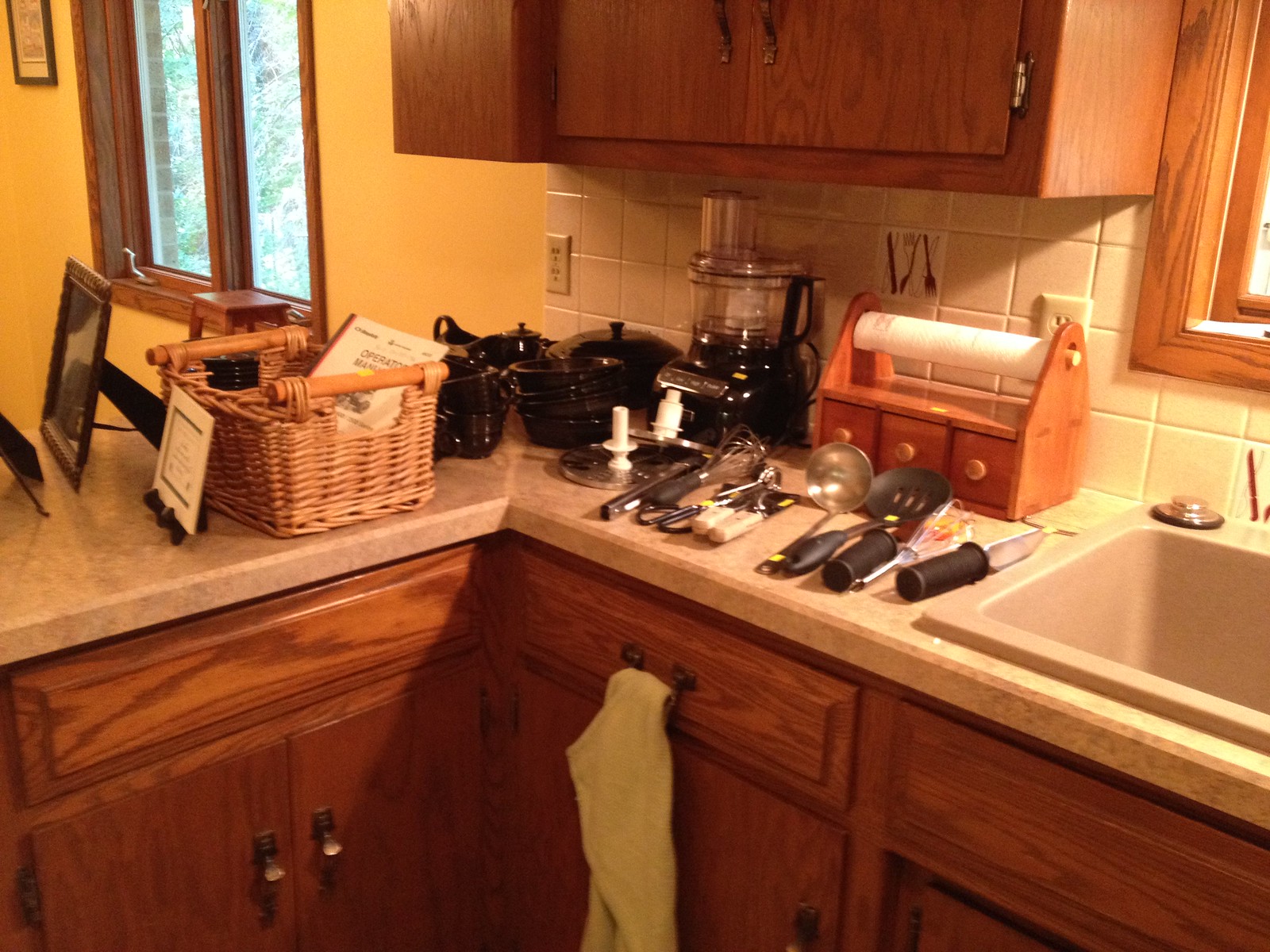The image depicts an L-shaped kitchen countertop, with the corner serving as the central point of the photo. To the left, a wicker basket sits on the countertop, containing a pamphlet and framed photographs, adding a touch of personal charm. To the right of the corner, a set of black pots and pans is neatly arranged, with a stack of bowls nearby. Further along the right side, various kitchen utensils are visible, including a ladle and a black plastic spoon with three cutouts. A blender is positioned against the wall, blending seamlessly into the background. The backsplash is adorned with white tiles, contributing to the kitchen's clean and bright ambiance. The upper cabinet, partially visible, hangs overhead, providing additional storage. On the far right, a sink equipped with a stopper is integrated into the countertop, completing the functional and organized kitchen space.